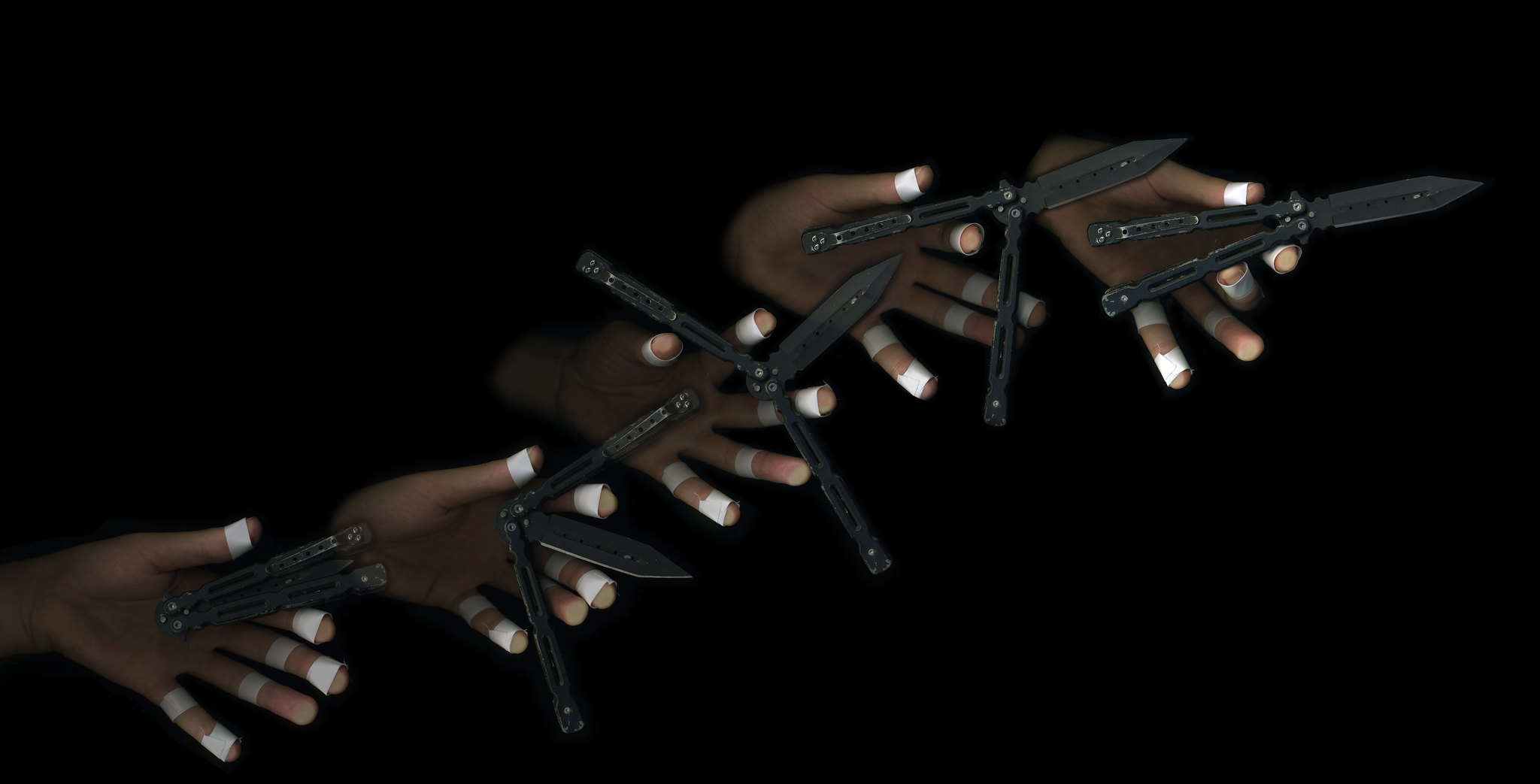In the dimly lit photograph with a black background, a series of five left hands, meticulously wrapped with white tape around the fingers, progressively demonstrate the unfolding of a folding pocket knife. The hands, arranged diagonally from the lower left to the upper right corner, hold the bronze-brown knife at various stages of its unfolding process. In the first image, the knife is completely folded, while in the subsequent images, it is gradually opened, with the final image showing the knife fully extended. The focus of the photo is sharply on the hands and the knife, with the background remaining in stark black, highlighting the step-by-step progression of the knife's transformation.